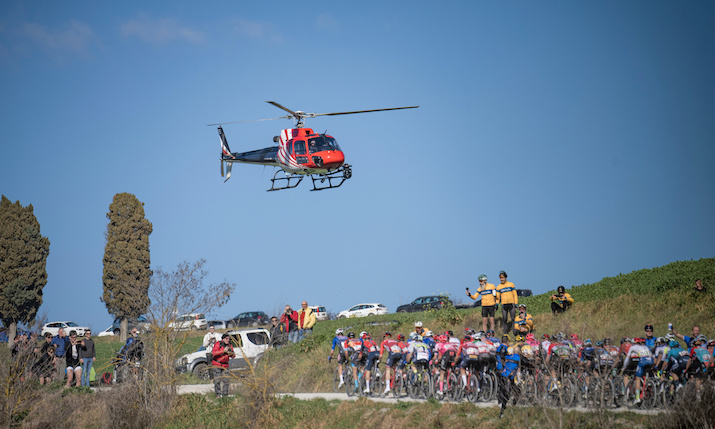The photograph captures a dynamic scene of a bicycle race taking place in a picturesque countryside setting. The narrow, one-lane gravel path is packed with a large group of cyclists, organized in a double file as they navigate a slight hill gradient. Above the racers, a red helicopter with distinctive red and white stripes near the engine and a black tail hovers approximately 60 feet in the air, likely capturing footage of the event against a backdrop of clear blue skies.

On the right side of the road, a green hill is dotted with spectators, some of whom are dressed in racing uniforms and are enthusiastically cheering on the cyclists. A team of four riders stands out, particularly one wearing a blue jersey. This group, along with other individuals scattered along the path, is actively photographing and filming the race. Tall, narrow trees line the path ahead, adding to the scenic countryside ambiance.

Towards the horizon, additional details emerge: a line of parked cars stretches along what appears to be another road, adding to the sense of a well-attended event. To the left, the landscape transitions into brambles, grass, and bushes, where more spectators and photographers are positioned, capturing the intensity and excitement of the race. An SUV or jeep can be seen further along, blending into the scene filled with energetic activity and vibrant colors.